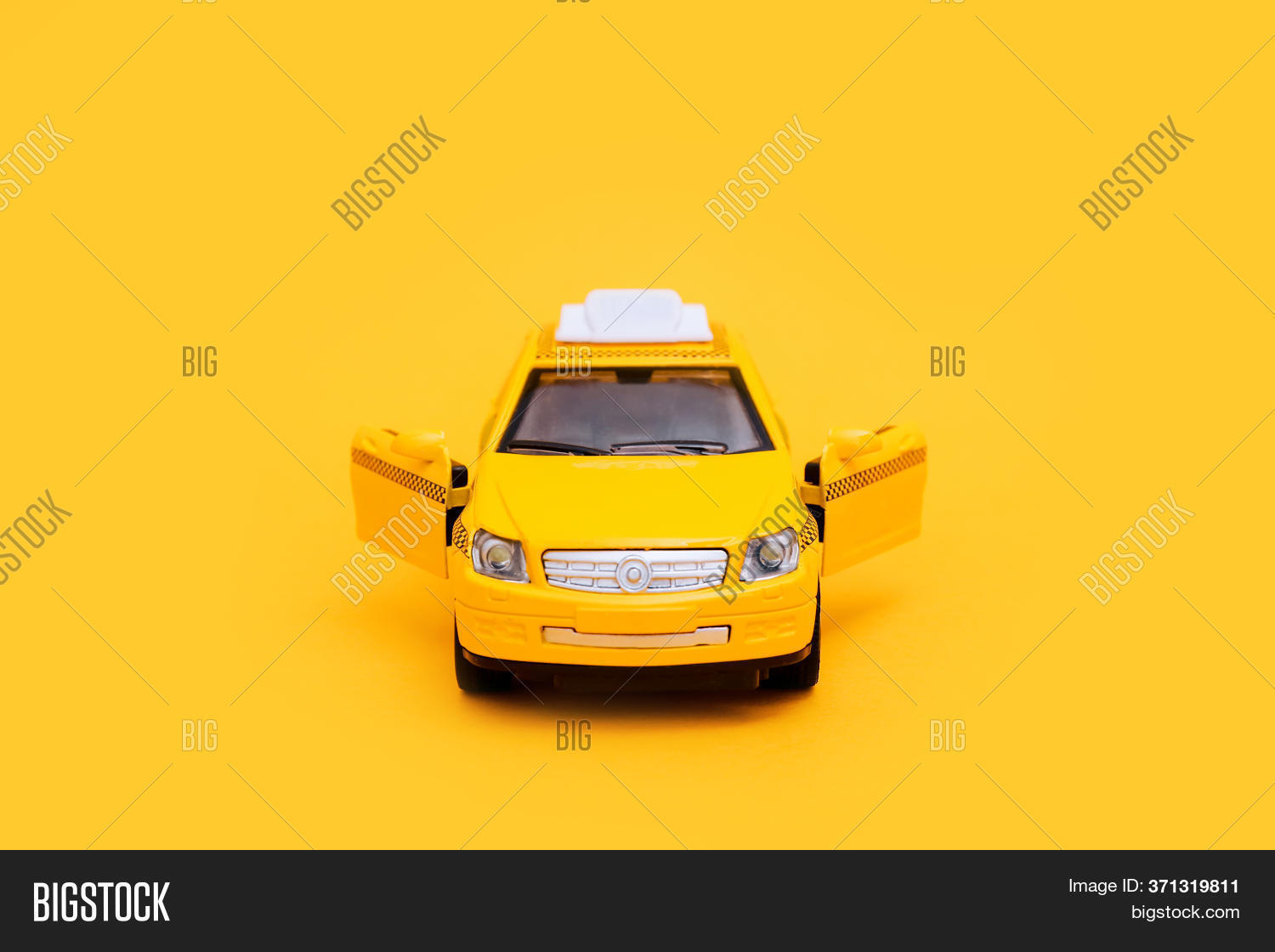The image is a rectangular combination of a photograph and digital creation, dominated by a bright yellow background. A black banner spans the bottom, displaying white text: “Big Stock” on the left, “image ID 371319811” on the right, and “bigstock.com” beneath. In the center of the yellow background is a yellow toy-like car, resembling a taxi with a rooftop sign area and brown stripes on the doors, which are both open. The car’s tinted windows and the somewhat angry expression formed by the arrangement of the headlights and grille add character. Overlaid across the image, "Big Stock" is repeated diagonally, indicating it's part of an ad campaign.